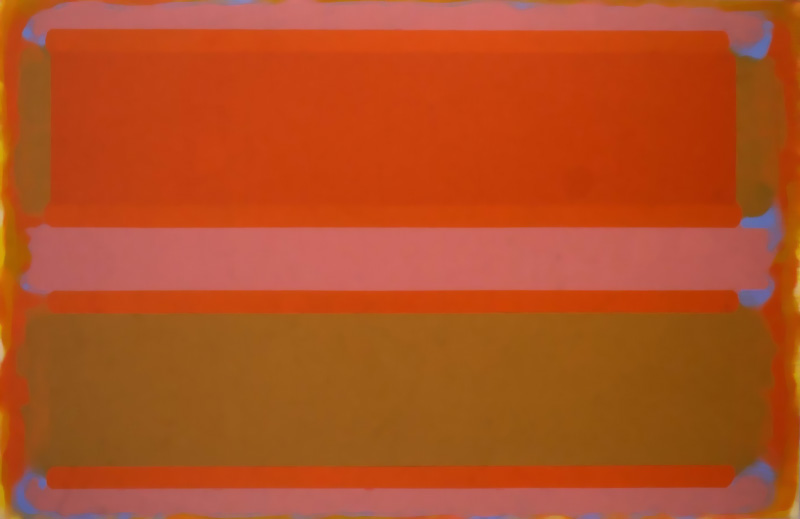This image depicts a modern abstract painting that is wider than it is tall, featuring a series of prominent horizontal lines of various colors and widths. Beginning at the top, there is a thin pink stripe, followed by a broad reddish-orange stripe with slightly lighter orange edging. Below this, a slightly narrower pink stripe is placed centrally, bordered by a dull peach stripe. Directly underneath the peach stripe is a wide band of beige or gold, capped at the bottom with another thin pink stripe. The painting has subtle blue detailing at the edges of these lines, which accentuates the otherwise dominant hues of pink and orange. The overall composition relies on the interplay of these vivid horizontal stripes, creating a balanced, yet vibrant aesthetic.